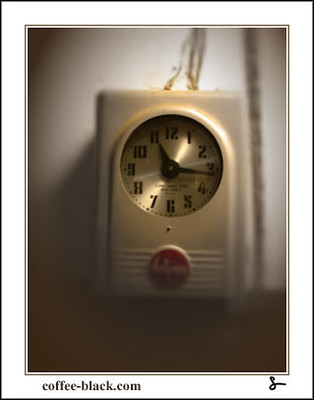A photograph with an outer white border features the website "coffee-black.com" printed in black at the bottom and a distinctive "S" shaped signature in the bottom right corner. Within this white border, the image is framed by a light brown margin, creating a vintage, sepia-toned effect at the bottom. The focal point is an off-white, plastic-cased clock adorned with wires extending from its top. The clock's face, silver in color, displays black numbers from 1 to 12, indicating the time as 11:16. Additionally, a red circle with unreadable white text is prominently displayed on the clock's surface.